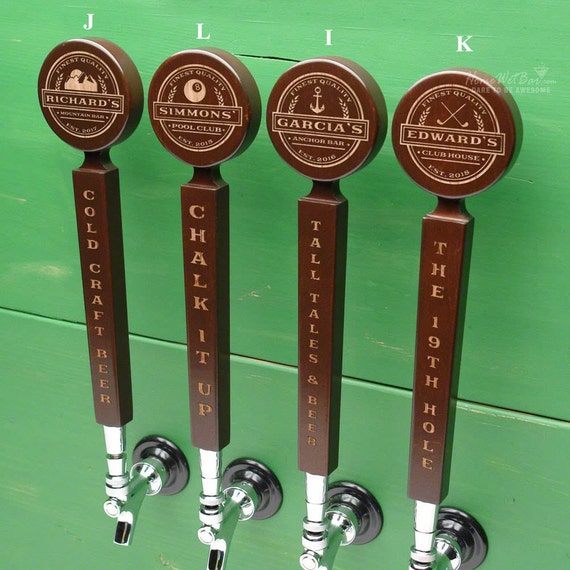This is a detailed photo of four beer tap handles, each with a distinct, yet similar design. The handles are mounted on a green painted wooden surface. The taps have square, tall handles topped with round, puck-like shapes featuring illustrations and names. From left to right, the taps are labeled "Richard's" with "Cold Craft Beer" inscribed vertically; "Simmons", which features a pool club theme with an eight-ball illustration and "Chalk It Up"; "Garcia's" with an anchor illustration and reads "Tall Tales and Beer"; and finally, "Edwards Clubhouse" with two crossed golf clubs and the phrase "The 19th Hole." Above each tap handle are white overlay letters, J, L, I, and K respectively. There’s also a barely noticeable watermark on the image, making it difficult to discern.